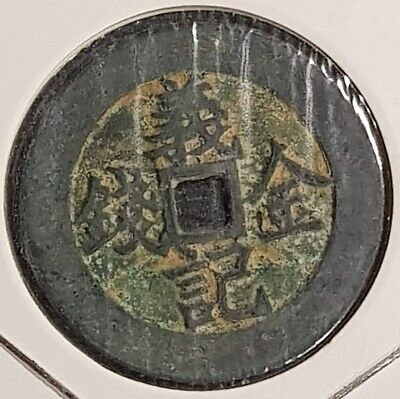In the center of the image lies a rare, round coin from the Qing Dynasty, dating back to the mid-1700s. This photograph showcases the coin resting on a white surface that features diagonal silver lines intersecting at various points. The coin itself has a distinct, dark bronze color with a grayish ring around its outer edge. Inside this ring, the coin's color transitions to a greenish-yellow bronze, with subtle hints of light brown. Prominent Asian characters adorn the coin at the top, bottom, left, and right positions, each character featuring a mix of curves, dashes, and horizontal lines.

At the coin's center is a prominent black square, encased within a slightly lighter gray square, emphasizing a contrast in shading. The entire coin appears to be shrink-wrapped in clear plastic, adding a sheen to its surface. This intricate and historically significant coin is the focal point of the photograph, positioned precisely in the middle of the white background, enhancing its detailed and preserved appearance in this representational realism style photograph.